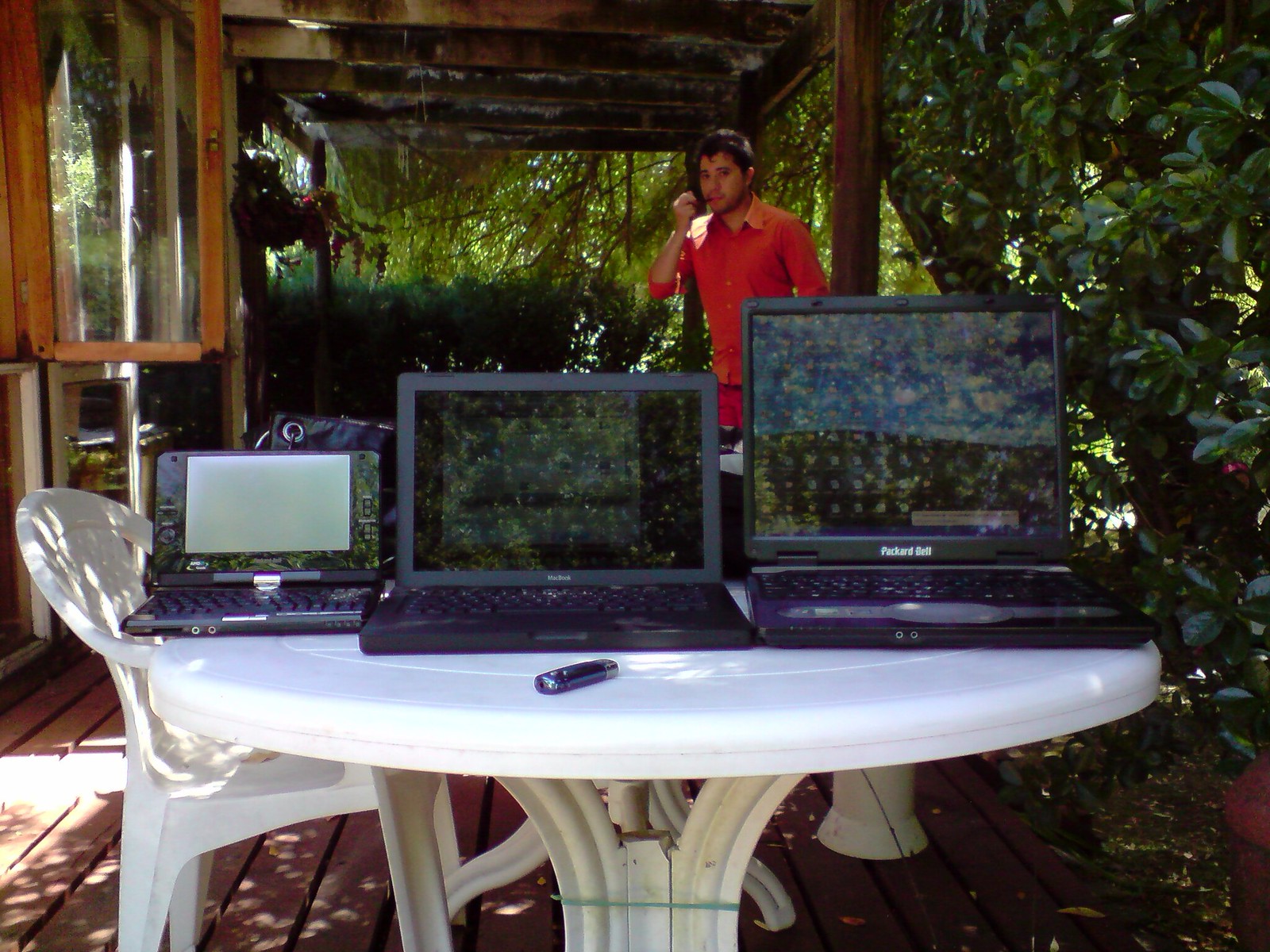The photograph captures an outdoor workspace, likely of someone working from home or a day trader, set on a redwood-style deck. Central to the image is a white table with a matching white chair to its left. Across the center of the table are three black laptops, arranged from the smallest on the left to the largest on the right. In front of the middle laptop lies a black cigarette lighter. To the right of the scene stands a man clad in a red button-down shirt and a headset with a microphone, adjusting it with his raised right hand. The background reveals heavy foliage and part of a pergola, indicating the deck is under a shaded overhang. The setting is lush with greenery, further enhancing the outdoor vibe of the workspace.